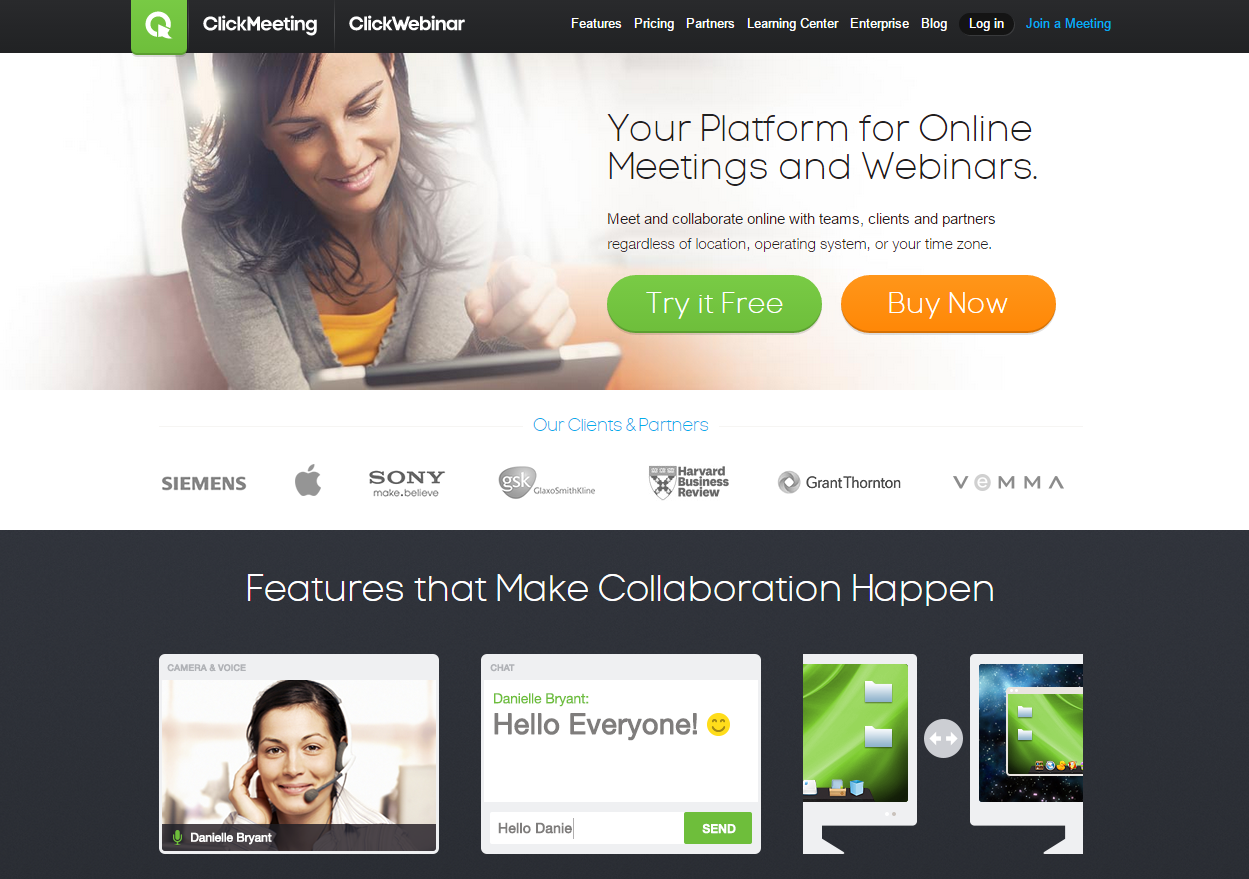### Descriptive Caption 

This screenshot features a webpage with a black top border containing a green square in the top left corner, which encloses a white circle with an arrow at the bottom. Adjacent to this icon, "ClickMeeting" and "ClickWebinar" are displayed in white font, followed by menu items: Features, Pricing, Partners, Learning Center, Enterprise, Blog, Login, and a "Join a Meeting" link in blue.

Below this header, an image showcases a woman with shoulder-length brown hair, wearing a long-sleeve gray shirt over an orange undershirt, engrossed in a tablet. The accompanying text reads: "Your Platform for Online Meetings and Webinars. Meet and collaborate online with teams, clients, and partners regardless of location, operating system, or your time zone." Underneath, two buttons are present: one green "Try it free" and one orange "Buy now."

Below this section, the gray-bordered area highlights the capabilities with the statement: "Features that make collaboration happen." Visual elements include a mock-up of Daniel Bryant's online presence, showing his camera and voice features, a chat interface where he says "Hello everyone," and images of two computer screens displayed side by side. Additionally, there is a list of notable clients and partners featuring logos of Simons, Apple, Sony, GSK, Harvard Business Review, Grant Thornton, and Vemma.